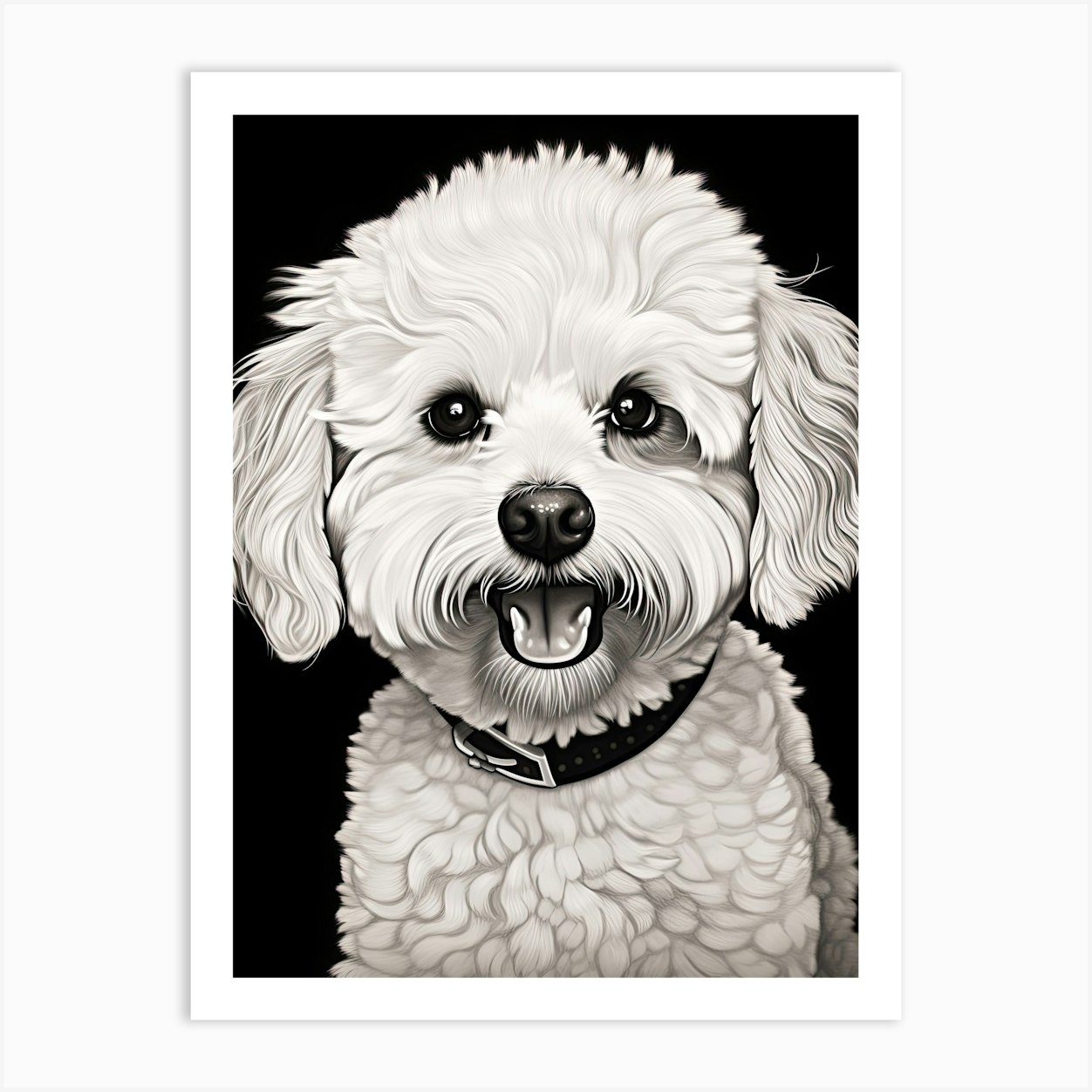In this detailed and highly rendered black-and-white illustration, a white, fluffy dog—resembling a Maltese poodle—takes center stage against a solid black gradient background. The creature's fur is meticulously depicted, with fluffy tufts around its head and body, and large, stringy ears that cascade downwards. The dog's round, black nose sits prominently above its open mouth, where its tongue and bottom canines are visible, giving the impression of a bright, cheerful smile. Its eyes are large, black, and shiny, reflecting light and adding liveliness to its expression. Adorning its neck is a black collar with a metal buckle, hinting at its well-cared-for status. The exquisite detail in the drawing, including the fine pencil lines that articulate the dog’s fur, and the clean, trimmed appearance, suggest the dog has been recently groomed. The image is striking in its simplicity and focus, with the white fur contrasting sharply against the black background, making the joyful dog the unmistakable focal point of the artwork.